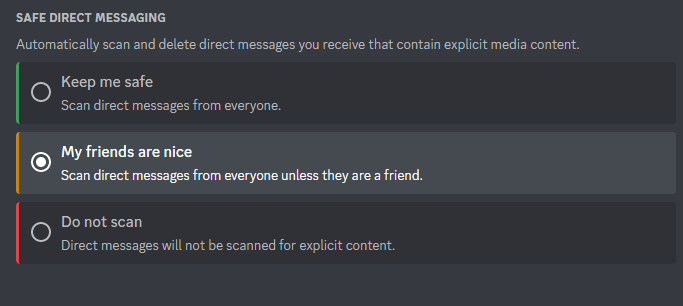This image is a screenshot from a website depicting options for safe direct messaging settings. At the top is a light black background with the title "SAFE DIRECT MESSAGING" written in bold, capitalized white text. Below the title, a descriptive line states, "Automatically scan and delete direct messages you receive that contain explicit media content."

Beneath this, there are three settings options, each within its own section and background shade:
1. The first option is on a darker black background with a green vertical stripe along the left side. It features a circular icon with a white perimeter and a black interior. The option text reads, "Keep Me Safe: Scan direct messages from everyone."
2. The second option, highlighted in a lighter black background, has a yellow vertical stripe on the left. The icon here has a white perimeter with a black outer ring and a smaller white circle in the center. The accompanying text states, "My Friends Are Nice: Scan direct messages from everyone unless they are a friend." This option is selected.
3. The third option is in a similar dark black background with a red vertical stripe. It also has a circular icon with only a white perimeter outline. The text for this option reads, "Do Not Scan: Direct messages will not be scanned for explicit content."

The image illustrates and emphasizes the safety measures available for managing direct messages with varying levels of scrutiny and privacy based on personal preference.